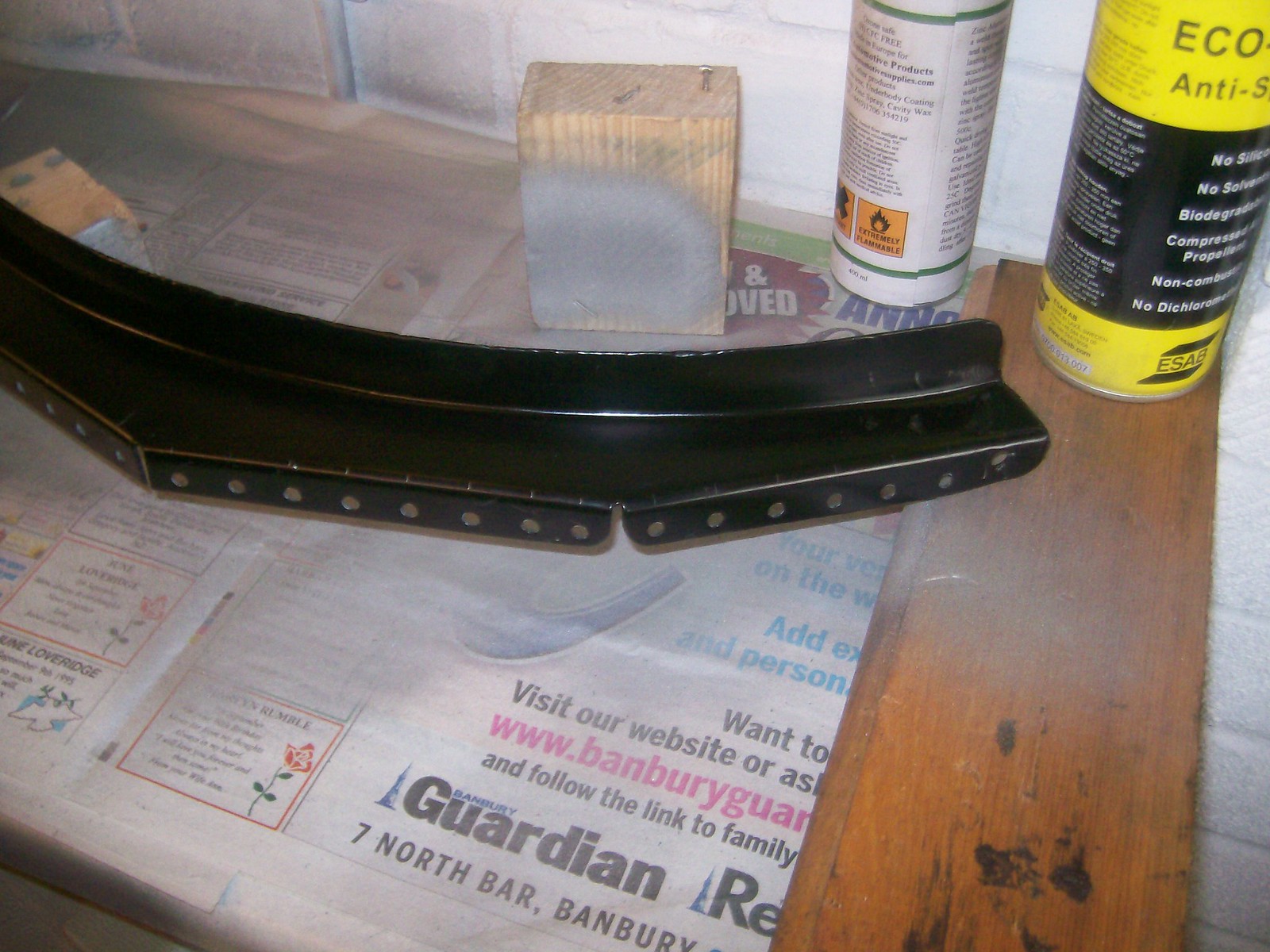The photograph features a black shiny metallic object adorned with silver dots situated on a piece of newspaper that covers a wooden surface. Behind this black metal piece is a light beige wooden block, possibly a small piece of 2x4, with silver paint sprayed on it. To the right, there is a yellow and black labeled tube, likely a paint can that reads "eco-anti-ESAB," and to its left, a white tube, which resembles a spray can. The newspaper beneath them has text that reads, "The Guardian 7 North Bar Banbury." For more information, visit our website at www.vanburygan.com or www.banburysomethinganother.com.